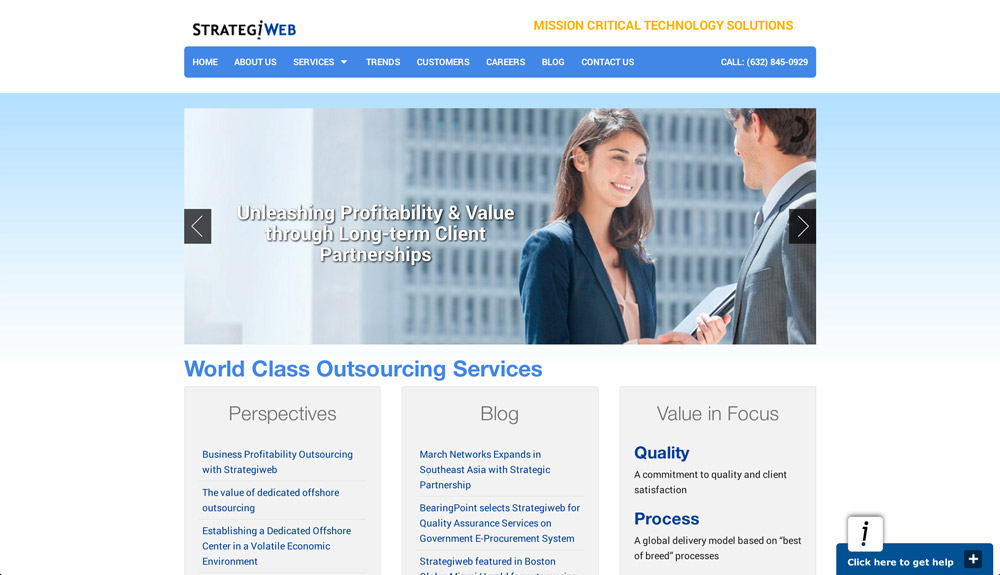Screenshot of StrategiaWeb Homepage

The screenshot captures the homepage of the website StrategiaWeb. StrategiaWeb is prominently displayed at the top with "Strategia" in black font and "Web" in blue. To the right of the logo is a tagline in yellow that reads, "Mission Critical Technology Solutions."

At the very top of the page is a blue navigation bar with the main menu items. Below this is a prominently placed image. On the left side of the image, text reads, "Unleashing Profitability and Value Through Long-Term Client Partnerships." 

The right side of the image features a friendly, professional scene: a smiling woman holding a folder engages in conversation with a man who is also smiling, suggesting collaboration and positive engagement.

Beneath the image, a bold blue text declares, "World-Class Outsourcing Services." A sub-menu follows this statement with three sections: Perspectives, Blog, and Value and Focus.

- Perspectives: Discusses various strategies to aid businesses.
- Blog: Covers current events and updates relevant to StrategiaWeb and the business world.
- Value and Focus: Emphasizes a promise of quality commitment and a global delivery model based on best practices.

This screenshot effectively highlights the core elements and navigation of the StrategiaWeb homepage, showcasing its commitment to technology solutions, client partnerships, and quality services.